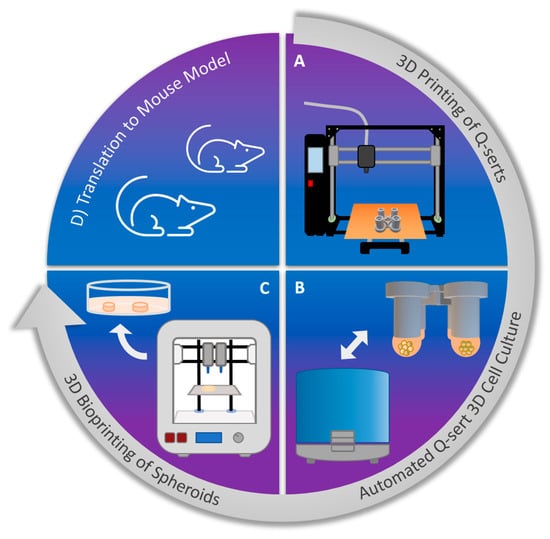This detailed educational illustration is highly stylized and likely intended for a textbook or scientific resource. Dominated by a blue circular shape, the image is segmented into four quadrants, labeled A, B, C, and D, with a gray border that features a directional arrow starting at the 12 o'clock position and ending at the 9 o'clock position. The overall design is rendered in shades of blue and purple with accents of black, white, and orange.

In Quadrant A, located in the upper right, there is a depiction of a 3D printing machine in black, with four spools positioned at the bottom. The text in this quadrant reads "3D printing of Q-CERTS." 

Quadrant B, the lower right section, showcases two items: one is a pair of cylindrical objects with orange-tipped ends, while the other is a turquoise cylinder. This quadrant's text emphasizes "Automated Q-CERT 3D cell culture."

Moving to Quadrant C, located in the lower left, there is an illustration of a petri dish containing two pill-like objects. This quadrant also features a schematic of a gray machine with two cylinders, two red buttons, a blue bar, and a brown dial. The text here indicates "3D bioprinting of spheroids."

Finally, Quadrant D, in the upper left corner, presents a simplistic white line drawing of two lab mice alongside the text "Translation to mouse model."

This meticulous representation provides a comprehensive visual overview of the processes involved in 3D bioprinting technology and its applications, marked by a clear and informative labeling system throughout each quadrant of the image.